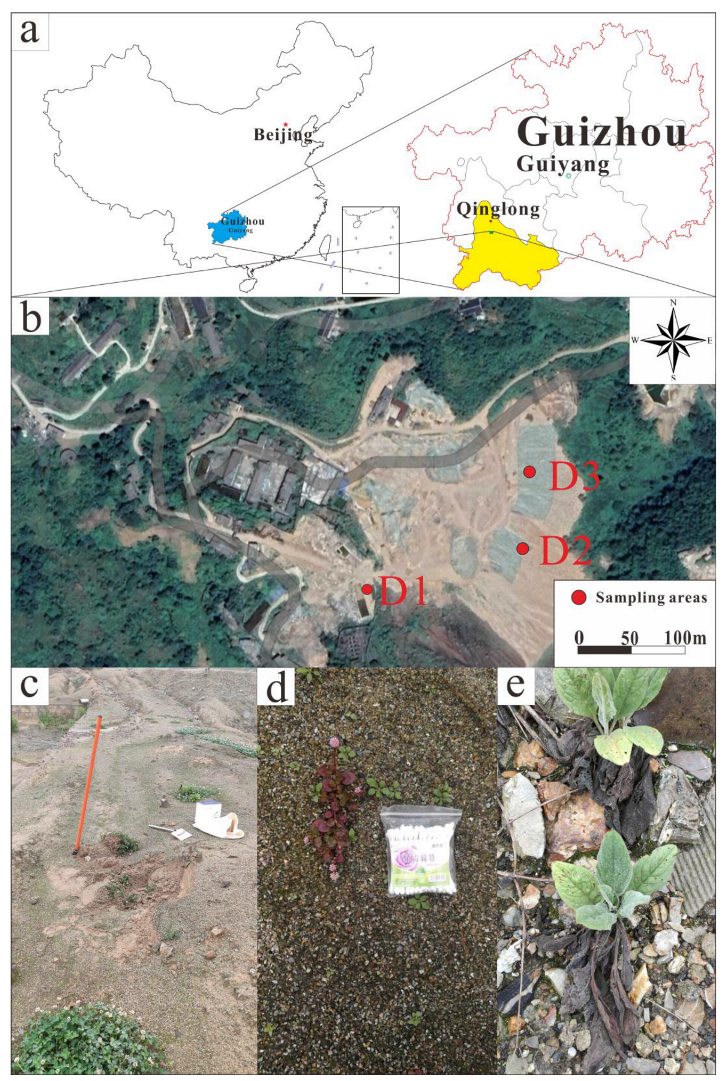This image is a multi-tiered graphic representation of a region in China, with various levels of detail focusing on specific sampling areas. The top section, labeled 'A,' is a simple, line-drawn map highlighting major cities like Beijing, Gaiyang, and Gaozhou, providing an overview of the region without delineating routes or streets. The next section, labeled 'B,' presents an overhead satellite view of the same area, marked with coordinates D1, D2, and D3, indicating sampling zones across the Northwest, East, and South to triangulate the layout. There is a scale bar indicating the sample areas' dimensions in meters. Below these, the image labeled 'C' shows a close-up of the ground marked by a red stick, suggesting the specific points of interest within the sampling zones. Image 'D' zooms further in to reveal a small Ziploc bag with white objects, indicating sampled materials. Finally, image 'E' captures the immediate environment of these sampled spots, showing the natural elements like dirt, rocks, and some vegetation, providing context to the sampling areas. It appears to be a detailed visual documentation for sampling purposes, possibly for a scientific or investigative study.